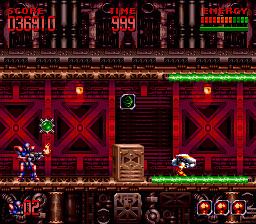This is a highly detailed screenshot from a video game, capturing a 1.5 by 1.5-inch portion of the screen. The image features a vibrant scene set on two levels or floors, distinguished by their colors and layout. In the upper right corner, the red score reads "036910," with the time set to "999" and the energy indicator showing four green segments out of a possible ten. Below this, there is a wall or a large box dividing the two central characters.

The character on the left, clad in a blue superhero outfit that obscures its face, appears to be armed with a gun that is emitting fire, indicated by a fiery effect at the barrel's end. His portion of the floor is brown with no green underneath. The character on the right is positioned on a bright green floor and seems to be bent over in pain. Above him, there is no green representing energy, indicating likely distress or injury.

The background features a wall adorned with purple and red "X" patterns. Additionally, in the lower right corner, there are three icons of small men wearing sunglasses, suggesting the player's remaining lives. The entire scene is set in a classic 2D side-scroller format, reminiscent of action or platformer games.